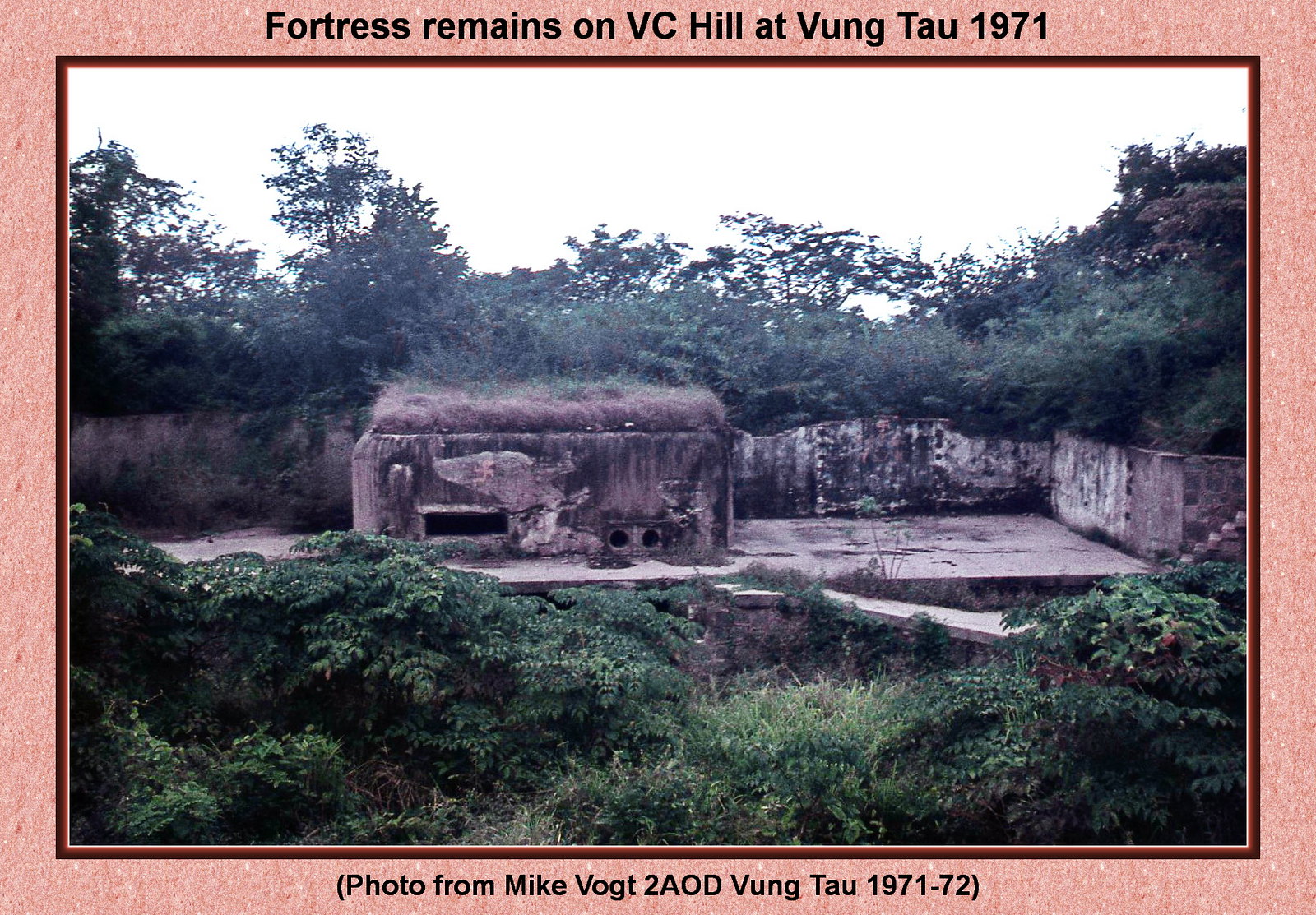The image, resembling a postcard and mounted on an orange card, depicts the deteriorated remains of a fortress on V.C. Hill at Vung Tau, Vietnam, photographed in 1971. At the top of the card, a caption reads, "Fortress Remains on V.C. Hill at Vung Tau, 1971," with a credit below stating, "Photo from Mike Vogt, 2 A.O.D., Vung Tau, 1971-72." The scene shows a stone platform, possibly a concrete slab, with the ruins of a stone structure. The fortress appears neglected and weathered, with grass and shrubbery encroaching upon and surrounding it. The stone structure has darkened, possibly from weather conditions, and displays a few round holes and a rectangular cut-out. A stone wall or concrete fence encloses the area, adding to the sense of abandonment and historical decay. The entire site is overrun with greenery, including trees, shrubs, and foliage, suggesting it hasn't been maintained over the years.